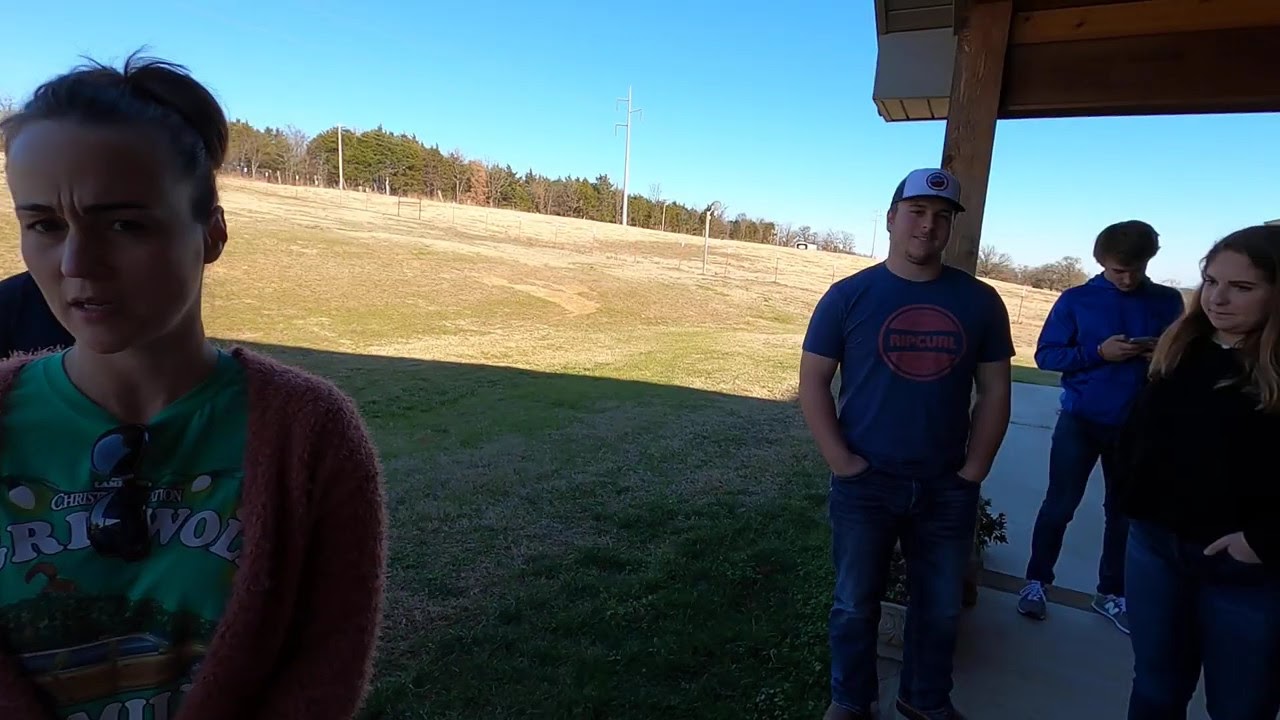This photograph captures a group of young adults standing casually under a wooden pavilion, located in a public park during daylight hours. The ground beneath the pavilion is made of gray concrete, while surrounding it is a grassy field, interspersed with some brown patches, and flanked by a distant tree line under a predominantly clear blue sky. In the scene's foreground, towards the bottom left corner, stands a dark-haired girl with her hair pulled back, wearing a green t-shirt partially obscured by an orangish, fuzzy cardigan, with black sunglasses anchored to her shirt. She appears to have her eyebrows furrowed. To her right, and further back, are more individuals, including a young man in a dark blue shirt and jeans, wearing a baseball cap and with his hands in his pockets. Next to him stands another girl dressed in a black sweater and blue jeans, her hands also in her pockets. Further right, another young man is captured looking down at his phone; he is dressed in blue and black. All individuals are casually dressed in attire such as t-shirts, sweaters, and sweatshirts, typifying the relaxed atmosphere of their gathering.